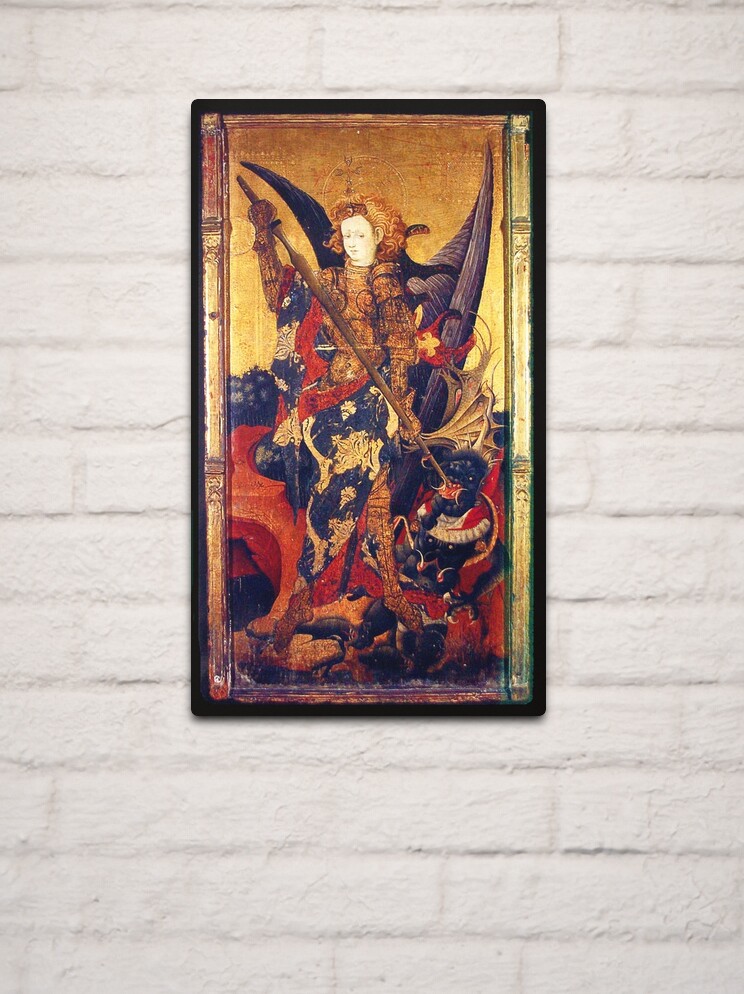The image depicts a highly detailed painting reminiscent of the 17th century, characterized by medieval or early Renaissance influences. The painting, framed in thin black, hangs on a white brick wall. It features a striking female warrior with long, golden-orange hair and pale skin, clad in golden-red armor. She wields a bronzed javelin or lance, which she appears to be using to strike a black and red, demonic-looking creature at the bottom of the painting. The background boasts a rich tapestry of golds, reds, and blacks, adding to the overall medieval ambiance. The vertically oriented artwork might suggest a depiction of a mythical hero, saint, or angel locked in combat with a beast, emphasizing a dramatic and heroic scene.